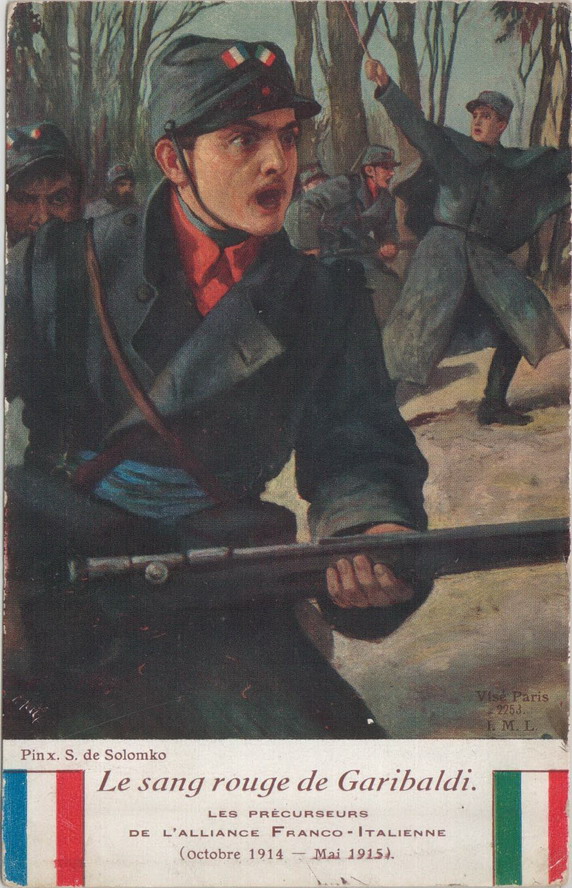The image is a richly detailed oil painting that serves as a piece of early 20th-century propaganda, possibly from the period between October 1914 and May 1915. The scene features a dynamically charged group of soldiers, predominantly characterized by their dark gray or blue overcoats and distinctive hats. Front and center is a male soldier in a dark gray overcoat adorned with a blue belt and wearing a red button-up shirt underneath. This central figure, who appears to be holding a rifle and possibly shouting, sports a hat decorated with both the French and Italian tricolor flags, symbolizing the Franco-Italian alliance.

In the background, additional soldiers similarly dressed in gray coats and caps can be seen, enhancing the sense of unity and shared purpose. The lower part of the painting includes a white banner with text and flags: the left side displays a tricolor flag with blue, white, and red stripes, while the right side shows a flag with green, white, and red stripes.

Multiple lines of text embellish the image, including the prominent words "Les Amg Rouge De Garibaldi,” a possible reference to Garibaldi's Red Shirts and their historical significance in the Franco-Italian alliance. The top of the image bears the initials P-I-N-X, S-D-E-S-O-L-O-M-K-O, suggesting the artist's signature or a dedication.